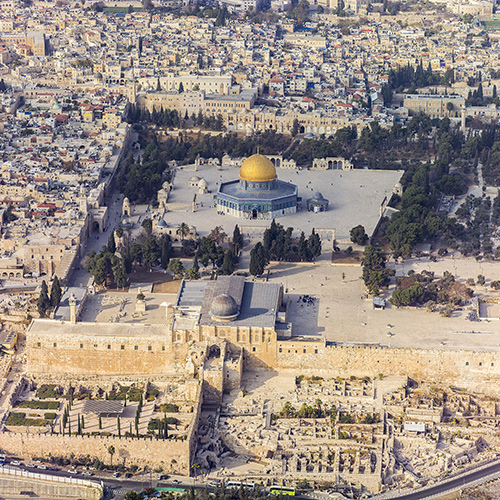This color aerial photograph captures an ancient desert city, possibly situated in the Middle East or India, showcasing its intricate architectural heritage. In the center of the image stands a prominent hexagonal building, distinguished by its large gold dome. The base of this building transitions from a dark blue hue to a pristine white as it meets the ground. Encircling this central structure are numerous older buildings, creating a near-wall-like formation around the dome. The area is dotted with several dark green leafy trees, providing contrast to the surrounding gray concrete and tightly packed old buildings, which dominate the left side and extend into the background. The foreground features light brown stone buildings that appear aged and weathered. The photograph, rectangular in shape, evokes a sense of history and cultural richness, with the central structure likely serving as a significant landmark or tourist attraction within the city.